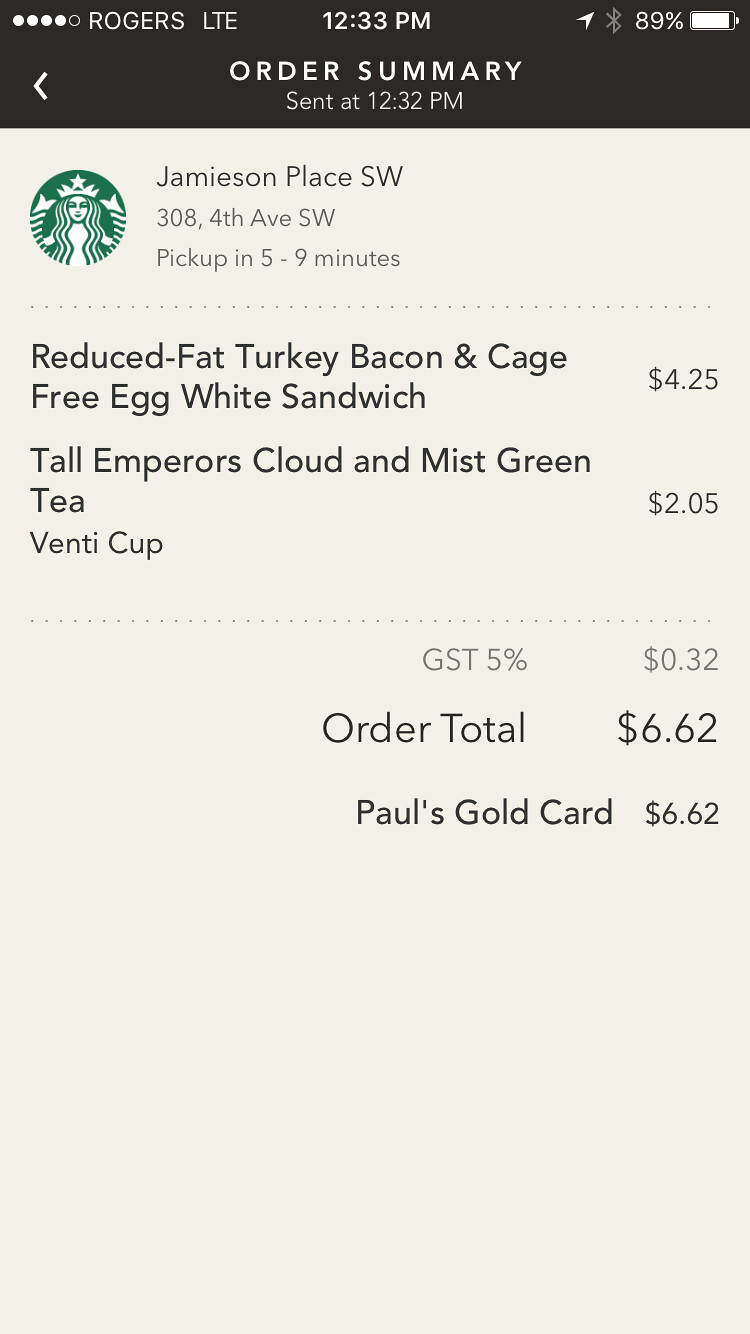This image appears to be a vertically aligned rectangular screenshot of a Starbucks receipt viewed on a smartphone. At the top, the status bar indicates "Rogers LTE" on the left with four out of five circles filled in white, showing a strong signal. In the center, the time is displayed as 12:33 p.m., and on the upper right, it shows an 89% battery life with a nearly full battery icon. Below the status bar, against a black background, it reads "Order Summary" and indicates that it was sent at 12:32 p.m.

Switching to a white background, the receipt features the Starbucks logo on the upper left, followed by the address "Jameson Place Southwest, 308 4th Ave Southwest". It notes that the order will be ready for pickup in five to nine minutes. A faint dotted line separates this header from the order details: 

First item: a "Reduced Fat Turkey Bacon and Cage-Free Egg White Sandwich" priced at $4.25,
Second item: a "Tall Emperor's Cloud and Mist Green Tea" in a venti cup priced at $2.05.

Another faint dotted line follows, leading to the tax breakdown: "GST 5%" amounting to 32 cents. The total order amount is listed as $6.62, paid via "Paul's Gold Card" with the same total of $6.62.

The lower part of the receipt is blank.